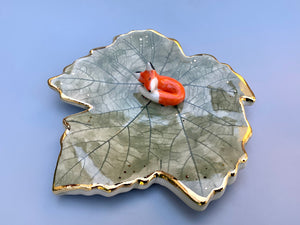This image features a decorative piece that resembles a leaf-shaped dish or ornament, crafted from enamel or porcelain with a glossy finish. The leaf is a pale green-gray or translucent bluish-gray, intricately designed with veins and trimmed in gold along its edges. Measuring about half an inch thick and possibly around six inches in length, the leaf rests against a pale blue background. At its center, where the veins converge, lies a small, intricately detailed ceramic or porcelain fox, curled up as if sleeping. The fox is approximately an inch long, with an orange-red body, white-tipped tail, and white fur under its jaw. It has black-tipped ears with white insides, and tiny black dots for eyes and a nose.